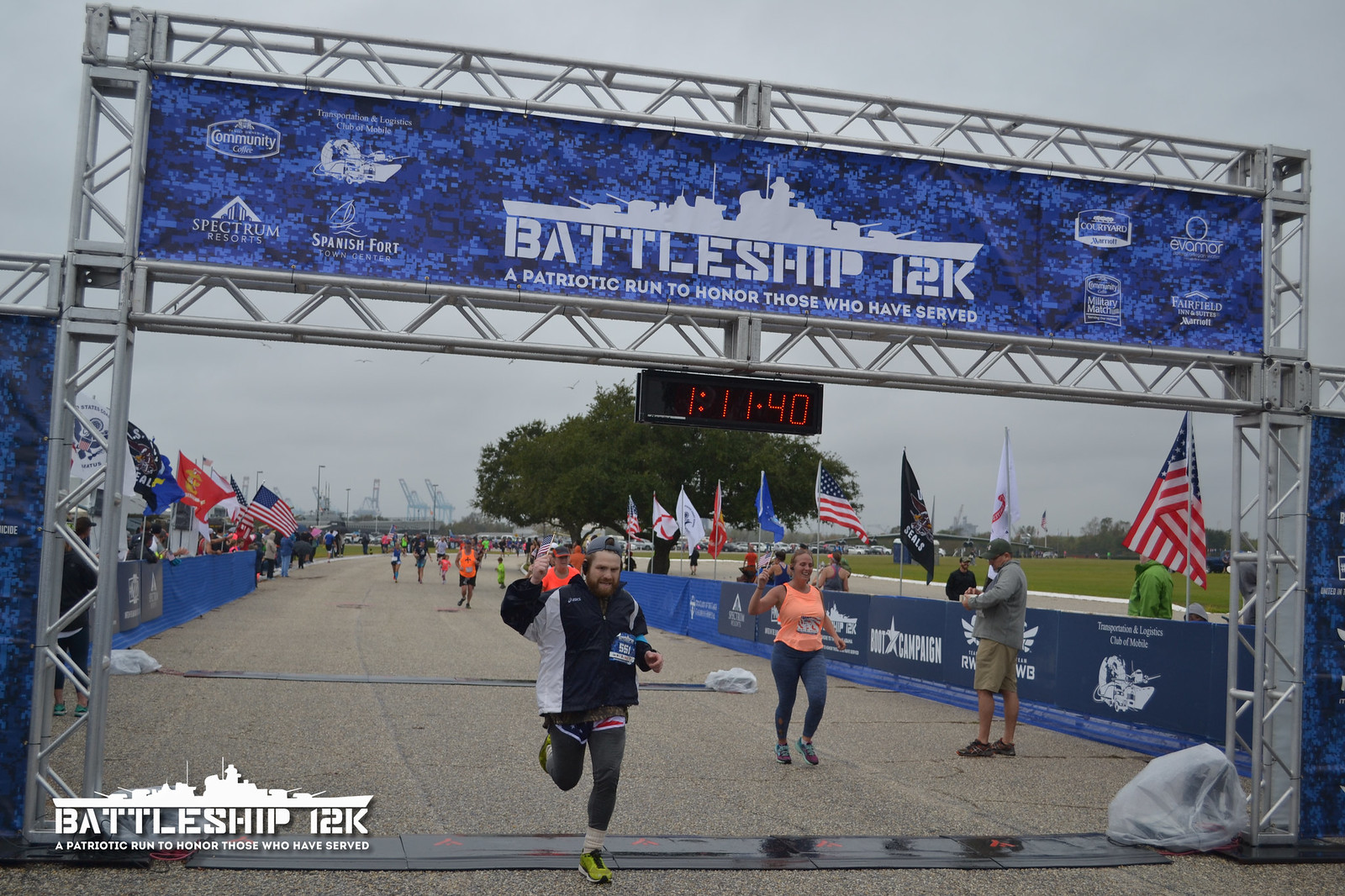A photo captures the dramatic finish of the Battleship 12K, a patriotic run to honor those who have served. Under overcast skies, a man in the foreground, wearing a backward gray hat, a black jacket, gray leggings, and lime green shoes, triumphantly crosses the finish line with his right fist raised high. Just behind him, a woman in peach-colored and gray leggings paired with an orange top is about to complete the race. The finish line is marked by a prominent silver archway draped with a blue banner that reads "Battleship 12K," featuring a hand-drawn silhouette of a battleship and the phrase "a patriotic run to honor those who have served." The banner also includes a clock displaying the time as 1:11:40 and flanked by white sponsor logos on either side. The course is lined with various flags, including U.S. flags and military banners, all set against a backdrop of blue barriers adorned with more sponsor logos. A man in a gray shirt can be seen snapping photos of the runners, while a long trail of other participants stretches behind, adding to the event's sense of scale and camaraderie.